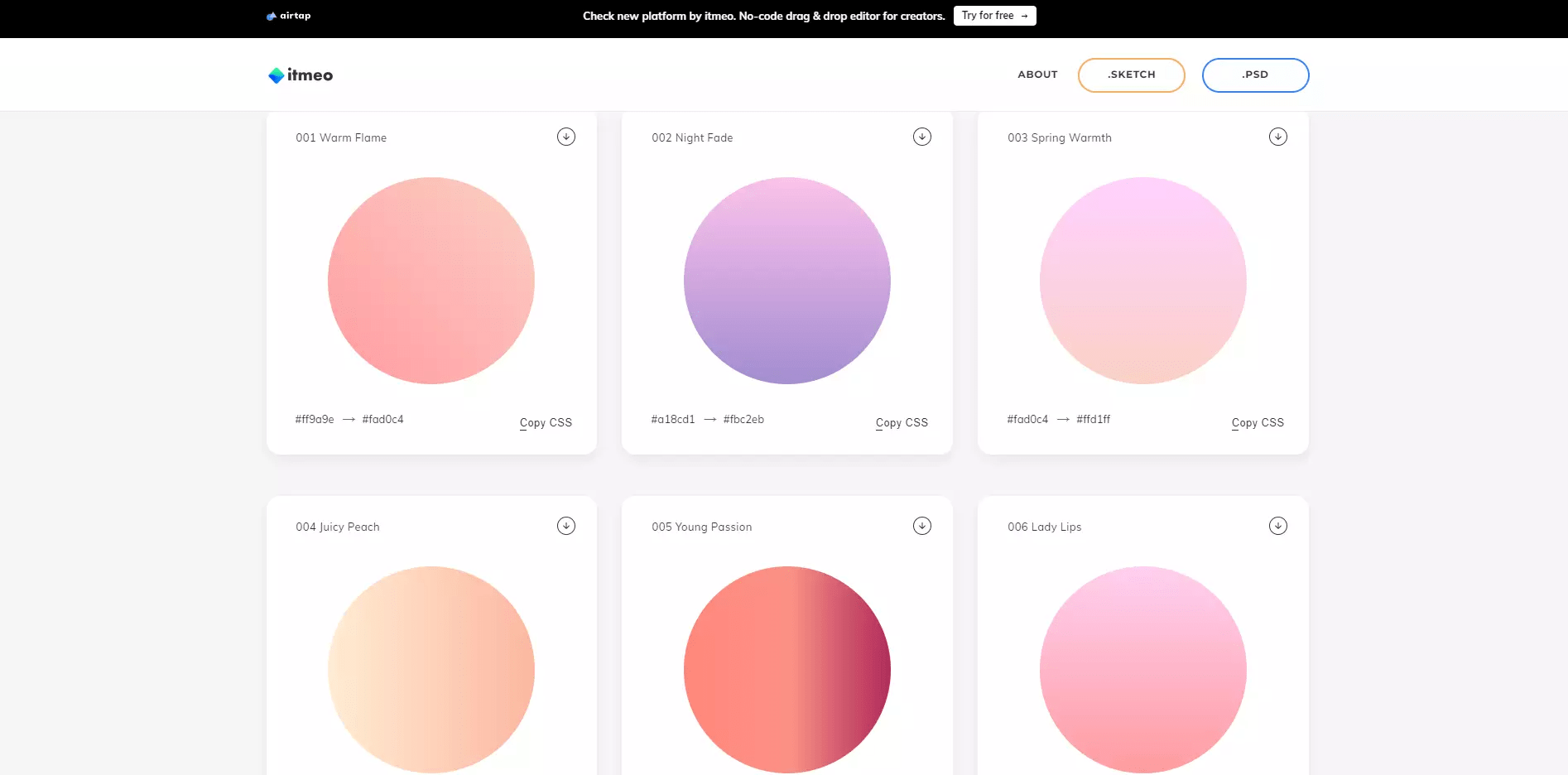The image depicts a webpage layout. In the top-left corner, there appears to be the website name, possibly "IMEO" or "ITMEO," accompanied by a logo icon. The top section of the page features a thin black banner with some hard-to-read text and a similar icon on the left side.

Prominently displayed in the middle section of the webpage is a call-to-action message that reads "Click New Platform, Buy," followed by additional indistinct information. Below this message is a rectangular box with a drop-down arrow and a "Try for Free" option.

Further down the page, there is an "About" section with two oval-shaped buttons next to it. On the left side of the section, six images are presented in boxes with rounded corners. Each box contains a circle filled with different shades of color. The first circle is a light peach color, the second is a light purple, the third is a pale pink, and the remaining circles follow a similar light color pattern.